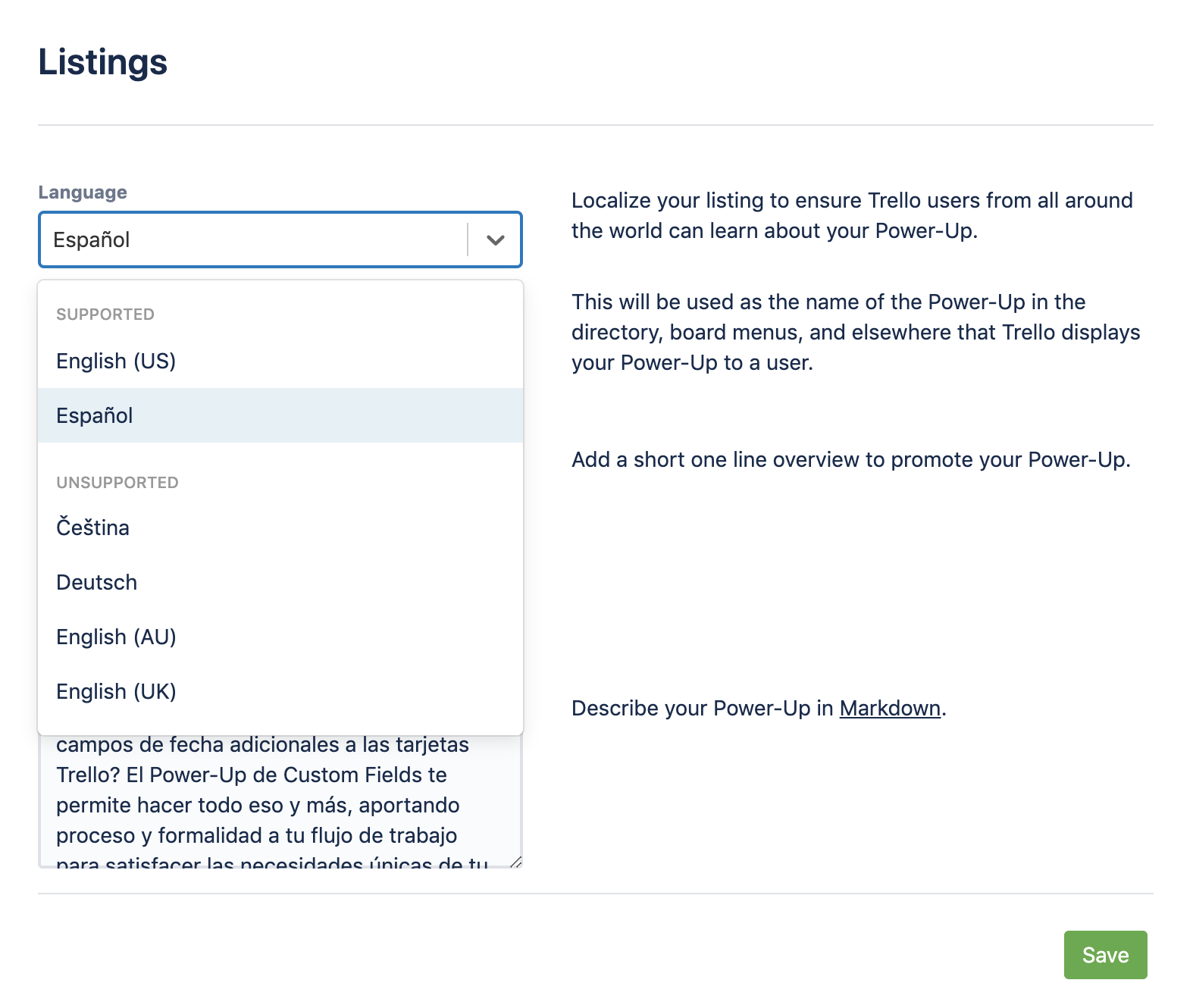This image is a horizontally oriented screenshot of a web page. The top left corner of the page is titled "Listings" in bold black font. Below the title, there is a left-hand sidebar labeled "Language." Inside this section, a blue highlighted box with a downward-pointing arrow displays the word "Español," indicating the currently selected language. 

Under the "Supported" subsection, the languages "English (US)" and "Español" are listed, with "Español" distinguished by a light blue border. Following this, the "Unsupported" subsection lists "ČEŠTINA," "DEUTSCH," "English (AU)," and "English (UK)" in parentheses. Beneath the language listings, there is additional text provided in Spanish.

On the right side of the image, there is a column featuring a description with the heading, "Localize your listing to ensure Trello users from all around the world can learn about your Power-Up." This text explains that the title will be used across various sections of Trello, including the directory and board menus, to identify the Power-Up to users.

Further down, a prompt requests adding a short one-line overview to promote the Power-Up. At the bottom of this right-hand column, there is an instruction to "Describe your Power-Up in Markdown," with the word "Markdown" underlined. Finally, in the bottom right-hand corner of the image, there is a green "Save" button with white text.